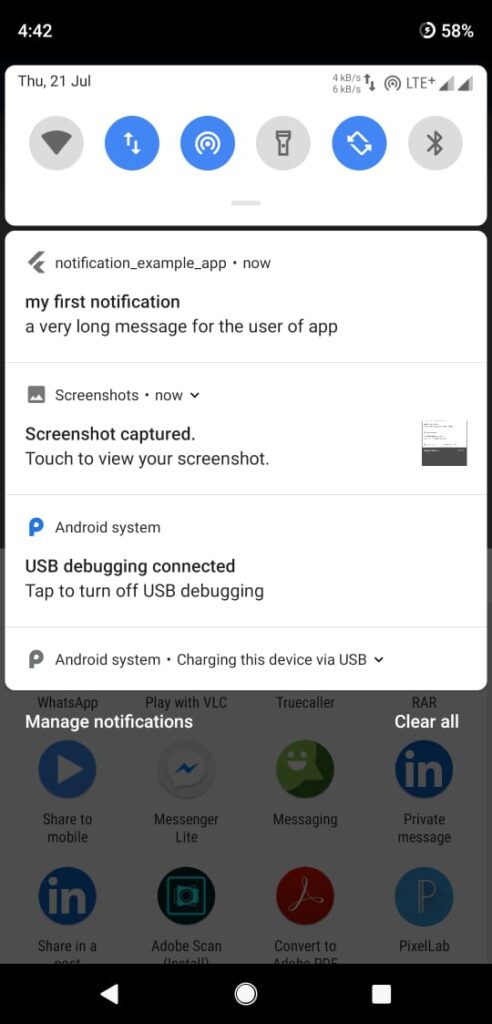Screenshot of an Android Phone with Active and Inactive Icons in the Notification Panel

This detailed screenshot captures the notification panel of an Android phone, offering a glimpse into both active and inactive system icons. Along the top row, some icons are active and highlighted in blue with white symbols, while others are greyed out, indicating their inactive status. The sequence begins with a WiFi symbol that is currently off, followed by an icon with two arrows pointing up and down, likely representing data transfer. Next, there is a target-like symbol with concentric circles, and then a greyed-out flashlight icon. Further along, an icon resembling a square with rotating arrows, which could be the tilt or auto-rotate function, is present. The Bluetooth icon is also greyed out, indicating it's not active.

Beneath these icons, the notification area reveals several alerts. The first notification is from an application, reading "Notification Example App Now," with an extended message indicative of a typical app alert. The second notification pertains to a screenshot, labeled "Screenshot captured, touch to view your screenshot," accompanied by a thumbnail preview on the right. The third notification concerns the system itself, stating "Android system USB debugging connected — Tap to turn off USB debugging."

Additionally, there is a persistent label indicating the device is "charging this device via USB," attributed to the Android system. Below these notifications, options for "Manage notifications" and "Clear all" are visible. In the semi-transparent background, several app icons for various services such as LinkedIn, Adobe PDF conversion, messaging, Pixel Lab, Share to Mobile, and Messenger Lite can be discerned, giving a broader context of the user's installed apps. This image encapsulates the typical layout and functionality of the notification panel on an Android device.